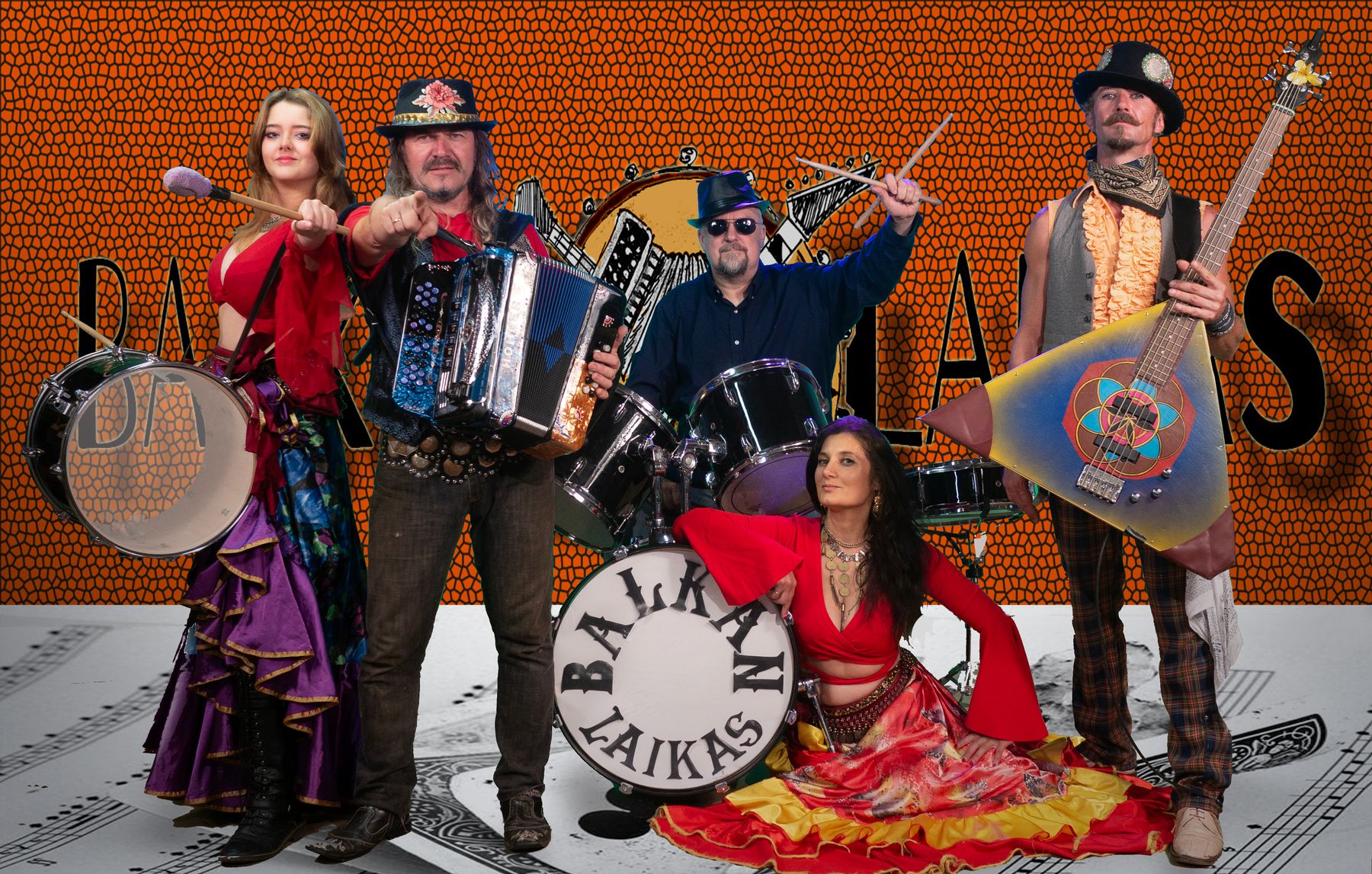This vibrant photograph captures the band Balkan Laikas standing against an orange, scale-patterned wall with obscured black text that also reads their band name. At the center bottom, a white bass drum prominently displays "Balkan Laikas" in black text. 

On the left side, a woman with blonde hair, pink lips, and a striking outfit comprising a red crop top and a purple skirt with blue accents holds a large, horizontally strapped drum. She gazes confidently at the camera, brandishing a drum mallet. 

Next to her, a man dressed in black jeans, a red shirt, and a leather vest with a black hat topped with a flower points towards the camera while holding an accordion in his left hand. 

In the middle background, a drummer dressed in black sunglasses, a dark hat, and a blue shirt holds two drumsticks crossed above his black drum set, which also bears the band's name.

Sitting in front of the drummer, another woman in a red crop top and a colorful skirt of yellow and red rests her arm on the bass drum, her long black hair cascading around her as she looks directly into the camera.

On the far right stands a man in dark plaid pants, tan shoes, a frilly pale orange shirt, and a sleeveless gray vest. He wears a black hat and a black-and-gold bandana around his neck, holding a large, colorful balalaika angled upward.

The band members, adorned in their eclectic and eye-catching outfits, seem to be advertising their dynamic presence and musical prowess.